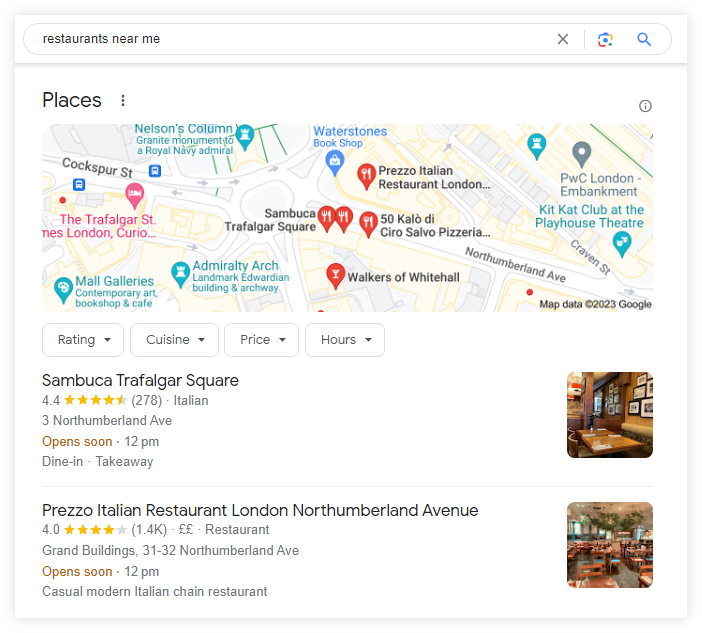The image captures a Google search result for "restaurants near me," displayed on a desktop screen. At the center of the screen is a map of London, pinpointed with locations of various establishments. Notably, landmarks such as the Kit Kat Club at the Playhouse Theatre, Trafalgar Square, Nelson's Column, Mall Galleries, and Admiralty Arch are marked in teal and gray, indicating entertainment venues rather than dining options.

Highlighted in red are several restaurants, giving viewers immediate suggestions. Among them:
- **Prezzo Italian Restaurant:** Located on Northumberland Avenue, London, this casual Italian chain restaurant has a rating of 4 stars and is set to open at noon. 
- **Sambacca, Trafalgar Square:** An Italian restaurant with a commendable rating of 4.5 stars, also opening at noon. A snippet includes a picture of a cozy booth inside the restaurant.

Additionally, the map indicates other restaurant options such as "50 Kilo D Ciro Salva Pizzeria" and "Walkers of White Wall."

Below the map, the image displays individual website links for each restaurant, allowing users to scroll for more detailed information about their dining choices.